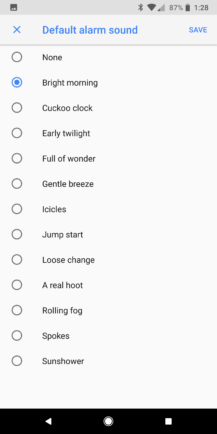A detailed screenshot of a color image shows someone's smartphone display at 1:28 PM, with the device's battery life at 87% and a full reception signal. The device has Bluetooth enabled. The top-left of the screen indicates currently running apps, with the image app being the visible one. The user is in a settings panel focused on alarm settings, shown prominently under the heading "Default Alarm Sound" in blue text against a white background.

The settings panel lists several alarm options: 
- None
- Bright Morning (currently selected)
- Cuckoo Clock
- Early Twilight
- Full of Wonder
- Gentle Breeze
- Icicles
- Jump Start
- Loose Change
- A Real Hoot
- Rolling Fog
- Spokes
- Sunflower

Options to go back or return to the home screen are available at the bottom of the display with tactile buttons labeled "Back" and "Home." This interface is straightforward and functional, dominated by blue and black text elements.